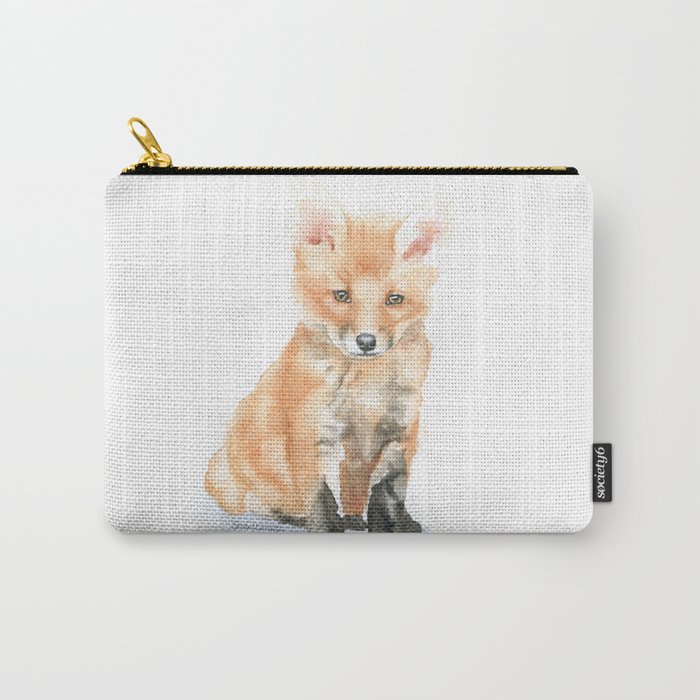This product image features a small, off-white coin pouch with a tweed texture. The central design on the pouch is a watercolor painting of a baby fox cub, sitting on its tail with its front legs positioned in front of it. The fox, rendered in rust brown with black paws and gray detailing on its front legs and shoulders, has green eyes, a black nose, and upright ears with pinkish interiors. The pouch is equipped with a gold metal zipper sewn into black fabric at the top. A small tag on the right side reads "Society6," indicating it is sold on a platform that features artwork from various artists. Photographed against a white background with a faint gray drop shadow, this detailed design makes the pouch suitable for holding small items, such as makeup or coins.